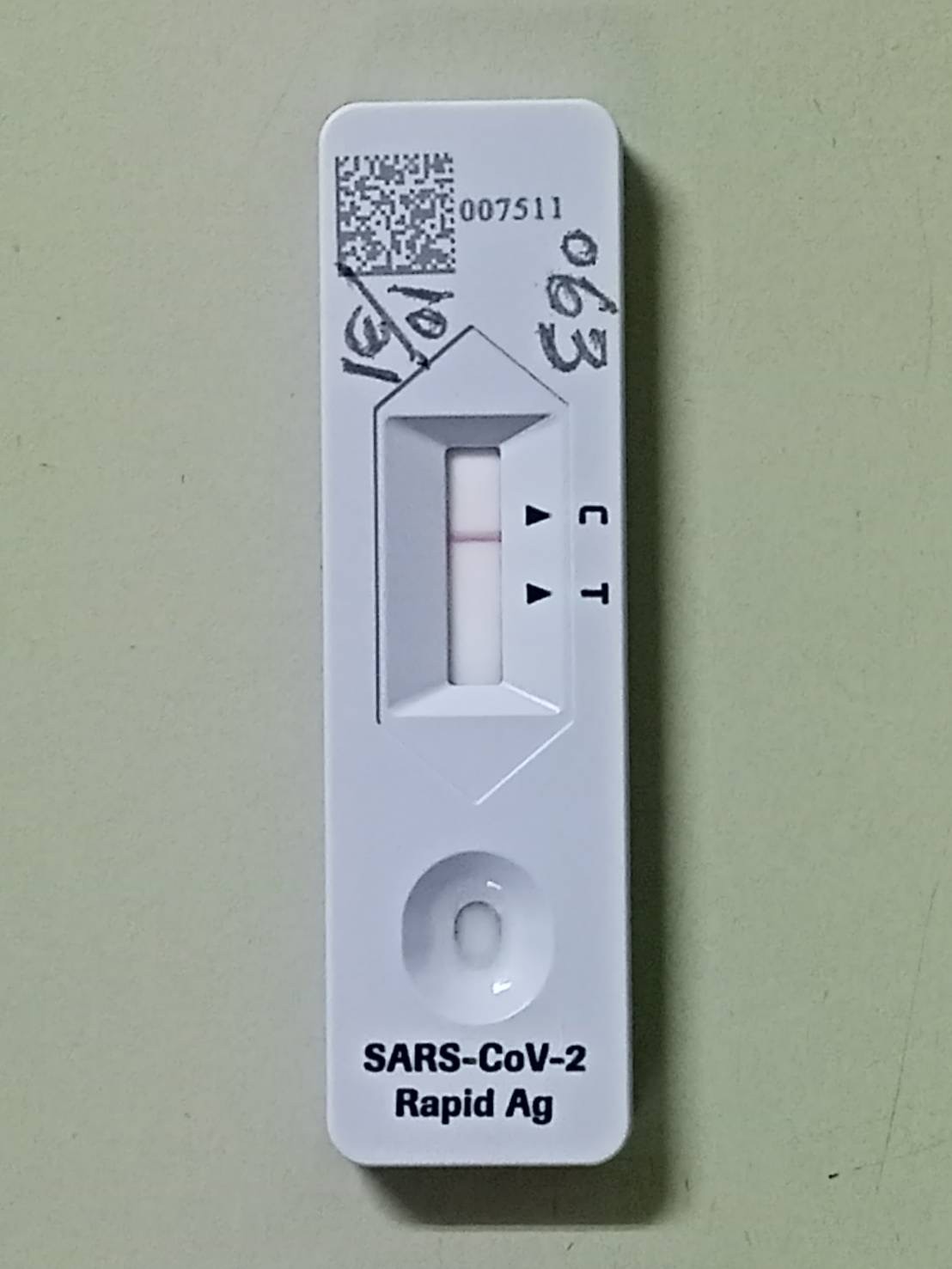This photograph captures a close-up view of a COVID-19 rapid antigen test placed on what appears to be an off-white medical lab countertop. The test kit, made of smooth, white rectangular plastic, stands vertically, reminiscent of a narrow tree trunk.

At the top left corner of the test, there is a small stamp resembling a QR code accompanied by the printed number sequence "007511." Handwritten on the right side of the test is the number "063," while "10/31," which likely signifies October 31st, is written on the left side.

Centrally located on the test is a window shaped like a house with a peaked roof. Within this window, a line has appeared on a white background, indicating the test results. To the right of the window are black arrows pointing to the letters "C" and "T," suggesting that the position of the line determines whether the result is a control (C) or test (T) result.

At the bottom of the test, there is a small well, possibly for placing the liquid sample to initiate the test. Beneath this well, the label "SARS-CoV-2" is printed, signifying that this is a rapid antigen test for detecting COVID-19.